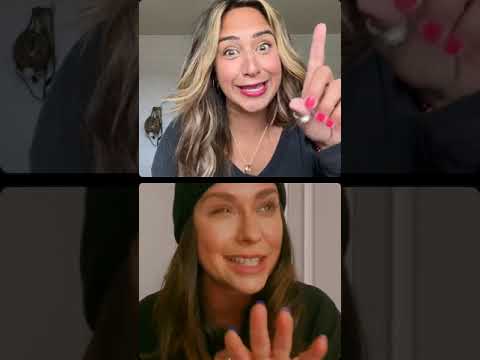The split-screen image features two women engaging in what appears to be a FaceTime conversation. Both women are smiling and looking toward the camera, giving an impression that they are enjoying their interaction. The image is divided into six squares, with the top and bottom central squares showcasing each woman, while the squares on the left and right magnify parts of their respective images.

The woman on top has a mix of blonde and streaked hair and is wearing a blue long-sleeve shirt. Her pink nail polish and lipstick add vibrant accents to her look. She sports a necklace with a ring pendant and is pointing up with her index finger. The background reveals a white wall adorned with a mask. On the sides, the left square enlarges her hair and part of the mask, while the right square highlights her hand and the sweater sleeve.

The woman in the bottom image sports long light-brown hair and a black stocking hat. She also has a large smile and a cheerful demeanor. Her fingernails are painted purple, and her palm faces up in her image. The left square shows a darker view of her long hair, while the right captures its opposite side against a white background.

Overall, the detailed description suggests a vibrant and happy conversation captured in split-screen photographs of two women, possibly indicating a friendly interaction or a moment of connection.